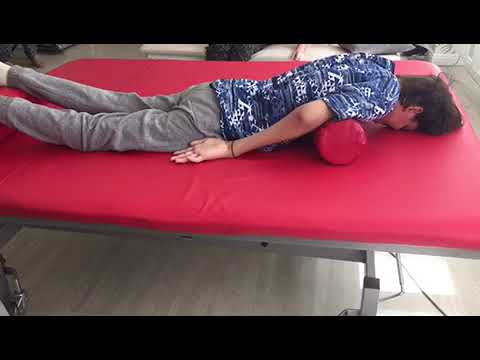In this indoor photograph, a man lies face down on a red mattress that appears to be part of a metallic veiled bed frame. Beneath his chest, serving as support, is a cylindrical pillow that matches the red color of the mattress. The man, with brownish-black hair, is dressed in a dark navy blue shirt adorned with white patterns resembling a Hawaiian or tribal design, and he wears gray jogging pants. His arms rest by his sides with palms facing up, and his legs extend straight back. The shiny, light gray synthetic floor beneath the bed contributes to the room's well-lit ambiance, suggesting it could be a gymnasium or a massage parlor. At the top and bottom edges of the image, horizontal black stripes are visible, adding to the room's structured appearance.